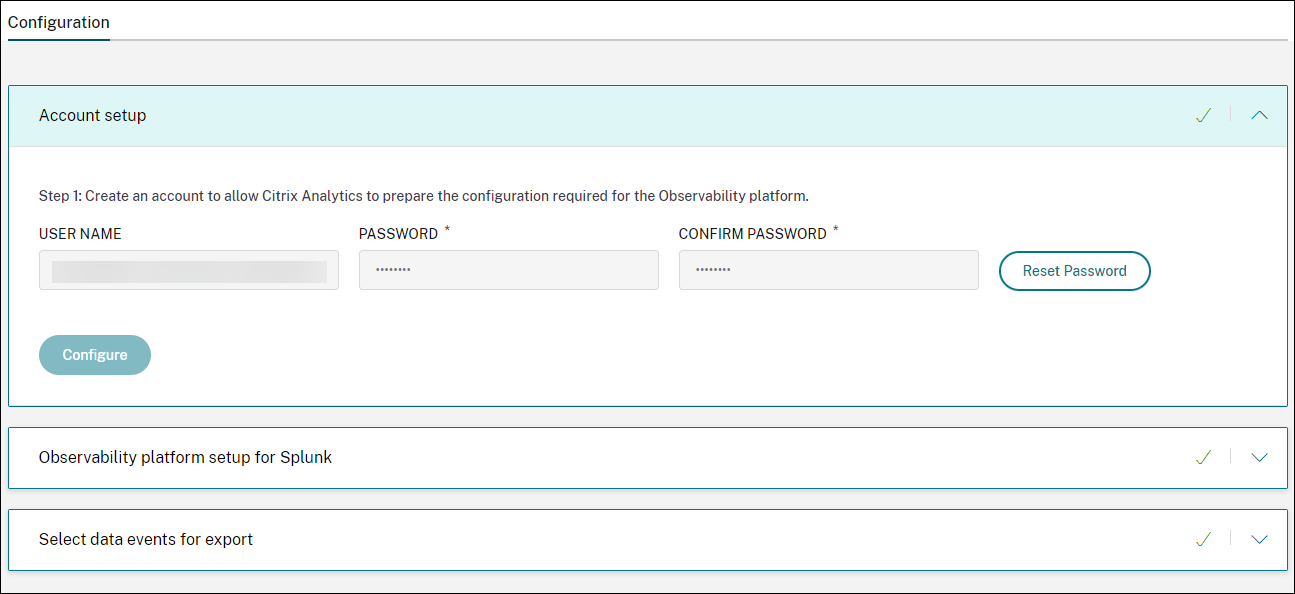This image is a detailed screenshot of a configuration page from a platform, potentially Splunk, identified through an on-screen mention. The page is specifically within the 'Configuration' tab, focusing on the 'Account Setup' section. 

In the 'Account Setup' area, Step 1 instructs users to create an account, enabling Citrix Analytics to prepare the necessary configuration for the observability platform. The form includes text boxes for 'Username,' 'Password,' and 'Confirm Password.' The 'Username' field is grayed out, ensuring anonymity, while the 'Password' and 'Confirm Password' fields are masked with asterisks to maintain security. Adjacent to these fields is a 'Reset Password' button.

Below this section, a notable light to dark blue-greenish 'Configure' button is present, inviting users to finalize the step. Further down, there is another setup section related to the observability platform for Splunk, which includes options to select data events for export. The page does not definitively confirm if it is for Splunk or another platform, but this gives a comprehensive overview of the current contents shown in the configuration tab.